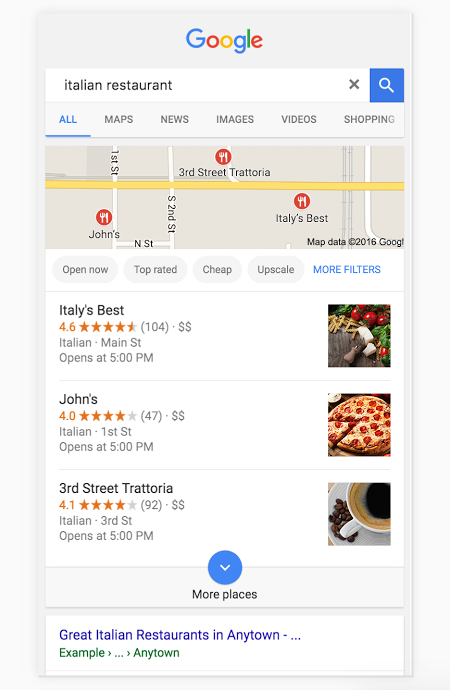The image represents a Google search for Italian restaurants. At the top of the page, the colorful Google logo is prominently displayed with its characteristic green, red, yellow, and blue letters. Below the logo, the search bar displays the query "Italian restaurant" in red text. The search results include a variety of options sorted by criteria such as "Open Now," "Top Rated," "Cheap," and "Upscale."

The first result is a restaurant named "Italy's Best," rated four and a half stars. It's located on Main Street and opens at 5 p.m. The accompanying image highlights a variety of vegetables, prominently tomatoes and some greens, suggesting a focus on fresh, vegetable-rich dishes.

The second result is "John's," which has a four-star rating and can be found on 1st Street. It also opens at 5 p.m. The image showcases a mouth-watering pepperoni pizza, emphasizing a classic Italian-American favorite.

The third result is "3rd Street Trattoria," also holding a four-star rating. It is situated on 3rd Street and opens at 5 p.m. The picture associated with this listing features a steaming cup of freshly ground coffee with coffee beans scattered around, hinting at their quality coffee offerings.

At the bottom of the search results, a blue circle labeled "More Places" with a downward arrow invites users to view additional options. Additionally, a generic suggestion prompts viewers to explore "great Italian restaurants in any town," providing a clickable link for further exploration.